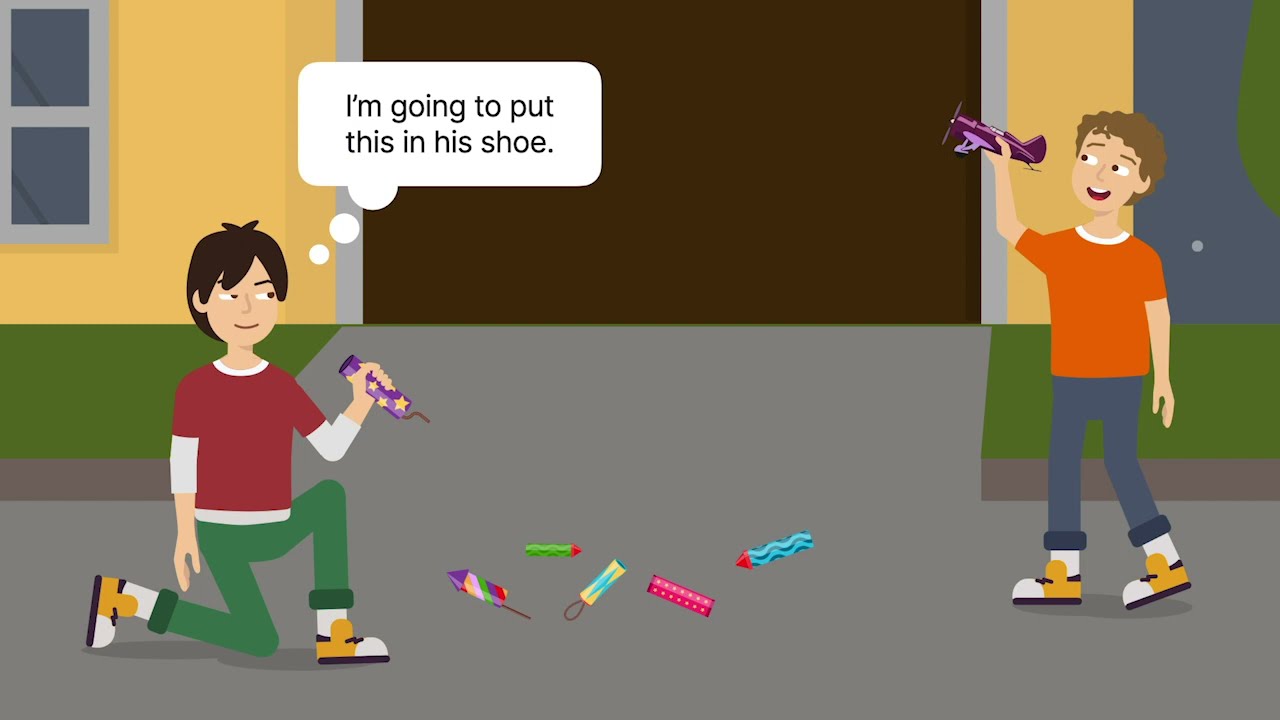The image is a detailed cartoon scene featuring two mischievous boys in a driveway in front of a yellow house with a brown garage door and gray window frames. The setting includes green grass flanking both sides of the gray driveway. 

On the left, a boy with short brown hair is kneeling on one knee. He is dressed in a red short-sleeved shirt layered over a white long-sleeved undershirt, green pants, and white and yellow shoes. He is holding a purple item with yellow stars in his left hand, which appears to be a firework. Above his head is a text bubble reading, "I'm going to put this in his shoe."

On the right side stands another boy with wavy brown hair, wearing an orange short-sleeved shirt, long dark gray pants, and white and yellow shoes. He holds a purple toy airplane in his right hand. Both boys are engaged in what appears to be a playful yet sneaky scenario, adding to the animated and lively nature of the illustration.